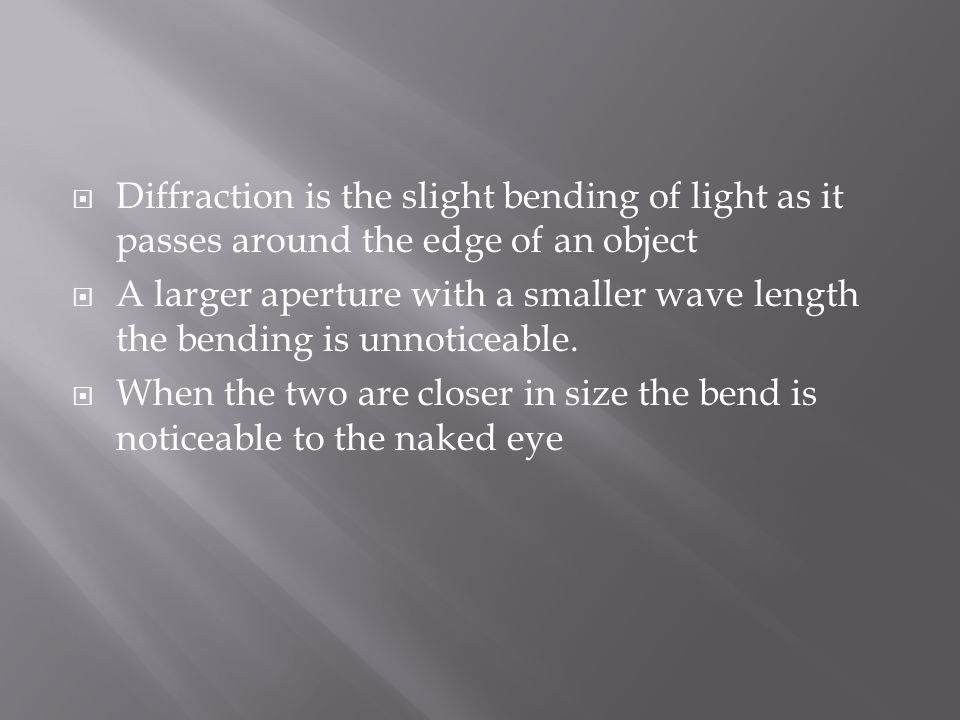The digitally created image features white text on a grey background, enhanced by a light effect emanating from the upper left corner. This light effect appears as rays extending diagonally across the image. The central content consists of three informational bullet points about the bending properties of light, known as diffraction. Each bullet point is prefaced by a white square outlined by another white cut-out square. The first bullet reads, "Diffraction is the slight bending of light as it passes around the edge of an object." The second states, "A larger aperture with a smaller wavelength, the bending is unnoticeable." The third explains, "When the two are closer in size, the bend is noticeable to the naked eye." This visual presentation underscores the principles of light diffraction and its effects.